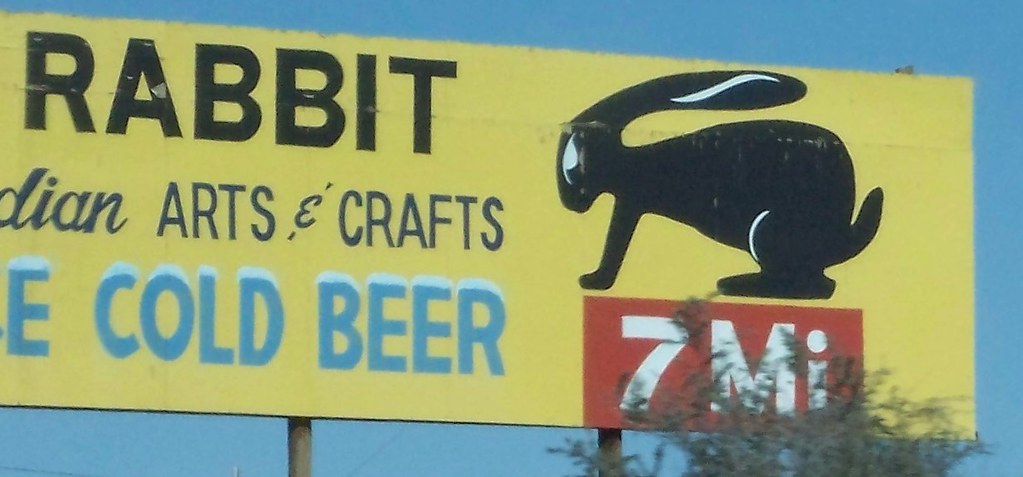The photograph captures an outdoor scene dominated by a partially visible billboard against a darker medium blue sky. The billboard features a bold yellow background with various elements in distinct colors. On the right side of the billboard, there is a stylized black rabbit outlined in white, crouched and poised, perched on a red block that reads "7MI." Below this, in black capital letters, the word "RABBIT" is prominent. Just beneath, in dark navy blue script, appears the fragmented word "DIAN," followed by more dark blue print reading "ARTS & CRAFTS." Further down, in a medium blue shade accented by white “ice” effects on top of each letter, the phrase "COLD BEER" appears, starting with a single capital "E" likely indicating the end of the word "ICE." The billboard is supported by visible poles and is set against a backdrop that includes the top of some trees, suggesting a rural American setting, hinting at an advertisement for a nearby convenience store or truck stop seven miles away.